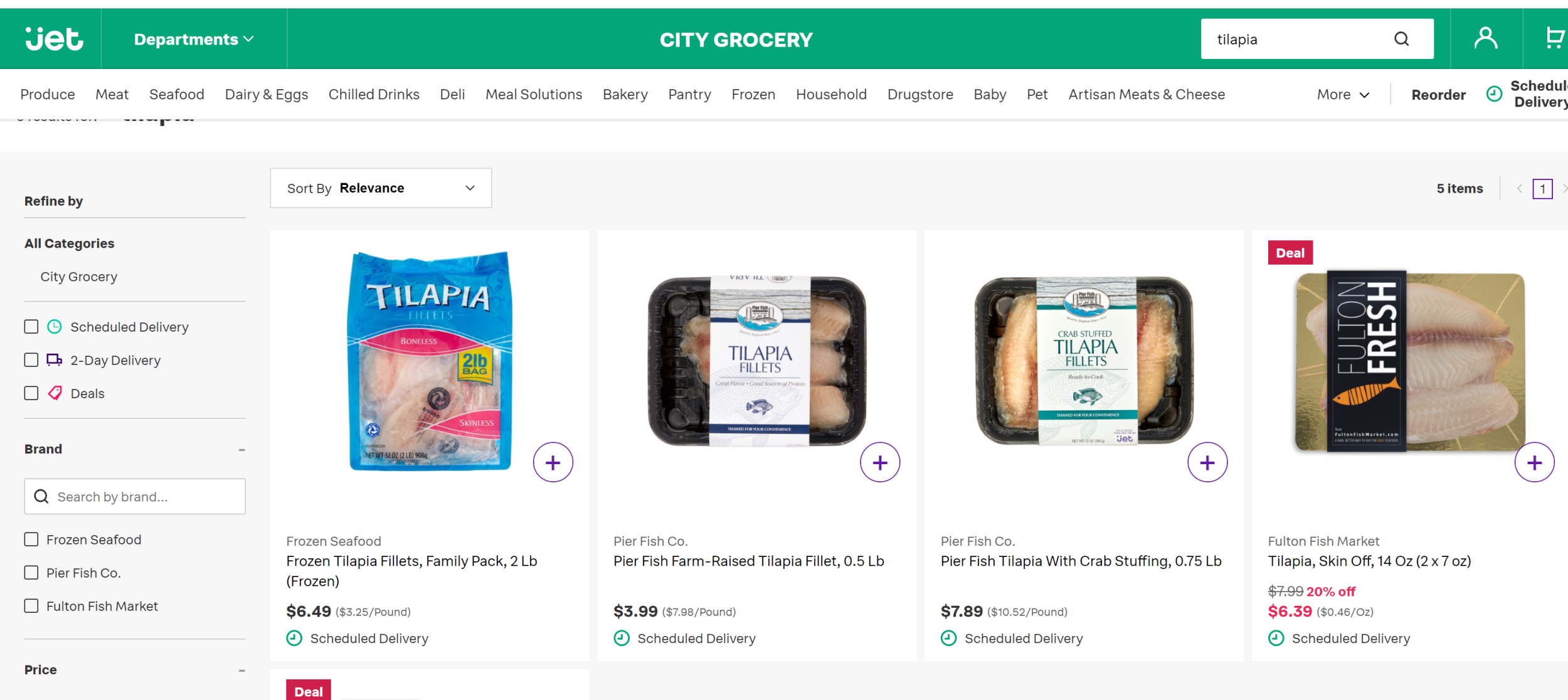This image depicts an online grocery shopping interface on a computer screen. At the top, a green banner prominently features the company's name, Jet, in the upper left-hand corner. The banner includes a drop-down menu labeled "Departments" and a search bar in the upper right-hand corner, where "tilapia" has been entered.

Below the green banner, a white navigation bar lists various grocery categories, including Produce, Meat, Seafood, Dairy & Eggs, and Chilled Drinks. Below this, a main content area displays four search results for tilapia. These include:

1. Frozen Tilapia Fillets, Family Pack, 2 lbs, priced at $6.49.
2. Pier Fish Company Farm-Raised Tilapia Fillet, 0.5 lb for $3.99.

On the left-hand side of the screen, additional search filters are available to refine the grocery selection. The interface suggests that shoppers are browsing and making purchases from an online grocery store, possibly called City Grocery, facilitated by the Jet app or platform. The context strongly indicates the user is specifically looking for tilapia options available for online purchase.